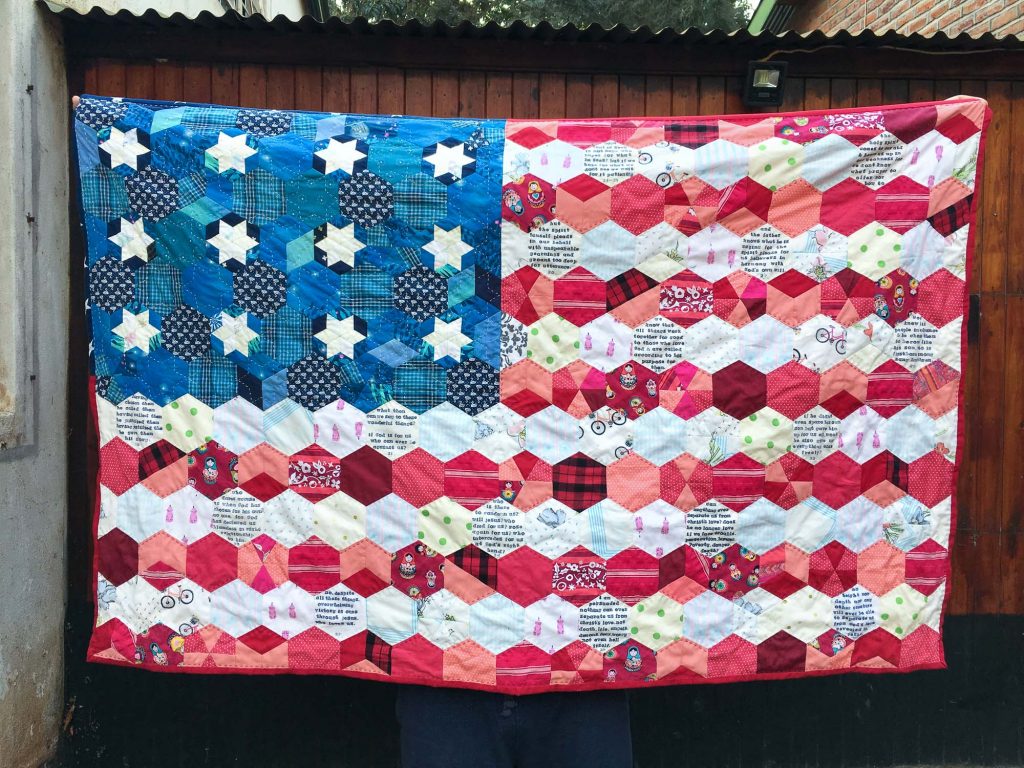This photograph captures a stunning quilt designed to represent the American flag, meticulously crafted from an array of small fabric pieces. The quilt's upper left corner showcases a field of blue adorned with stylized, large white stars arranged in three rows. Notably, the stars are not the traditional 50 but a dozen, each made from different shades of blue fabrics, including turquoise, bright blue, and navy blue with white patterns.

The remainder of the quilt is composed of alternating red and white stripes. Each stripe consists of diverse fabric panels featuring a variety of patterns, including stripes, plaids, floral designs, animals, bicycles, and even text. These fabrics range in intensity, with some square patches introducing subtle hues and others presenting bold motifs like scotch plaid and paisley prints.

The quilt is displayed outdoors, draped over a tall wooden fence. The eclectic mix of fabric styles and colors, combined with the iconic American flag design, creates a visually striking and uniquely beautiful piece of artistry.